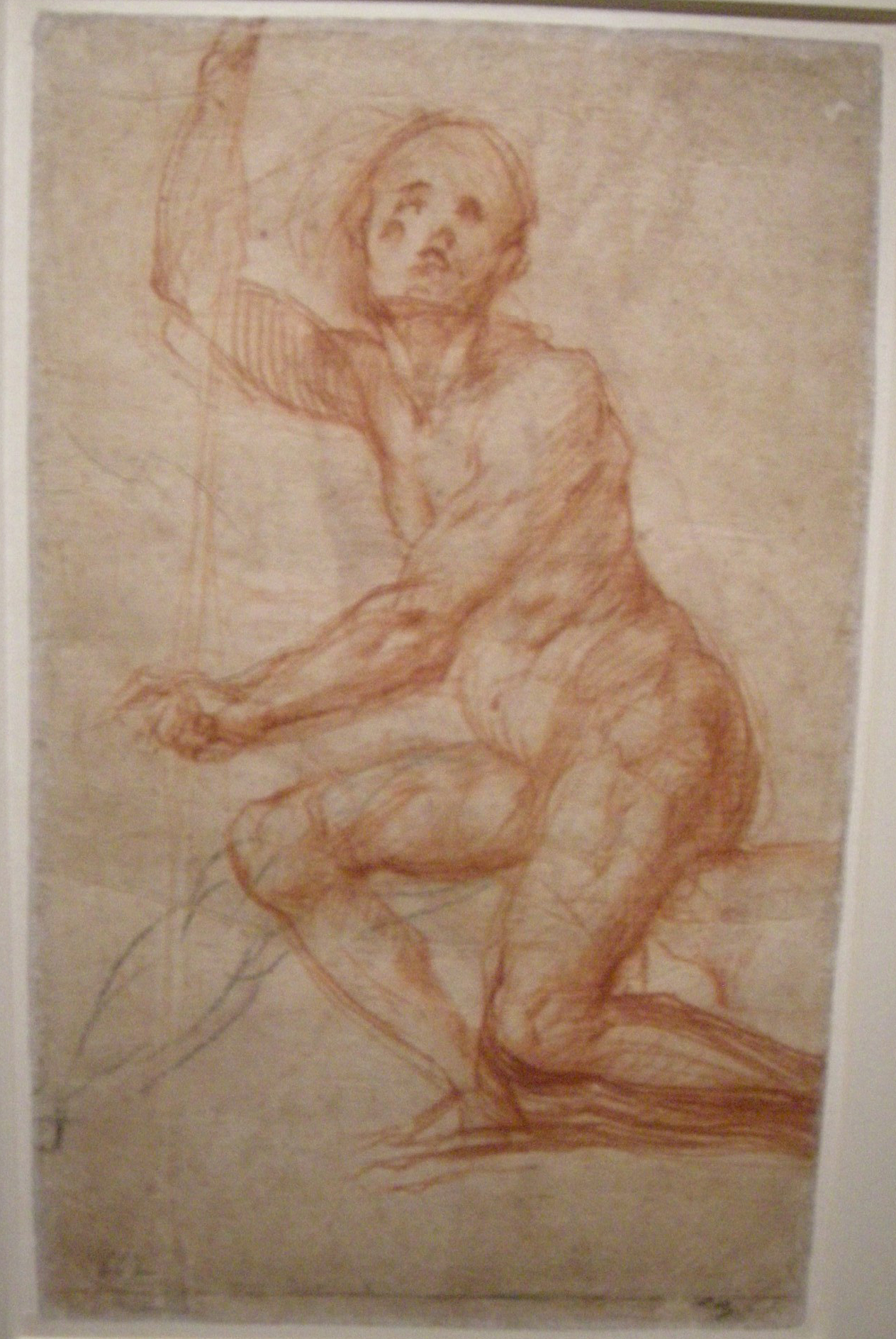The image depicts a detailed and textured pencil sketch of a muscular, unclothed human figure kneeling on the ground. The figure, drawn primarily in brown and orange hues, displays an intricate anatomical structure with pronounced muscles and bony features. The head is facing upwards and outward with a blank expression, marked by distinct facial features, including birthmarks. The left and right arms are extended, holding onto a thin, light-colored pole, giving an impression as if the person might be rowing or in motion. The body shows a slight roundness in the belly area, and the legs are positioned to the side. The background of the sketch is a brownish-tan color, accentuated with folds and textures, all set against a white backdrop. The entire image appears slightly blurry, adding to the artistic and vintage feel of the drawing.